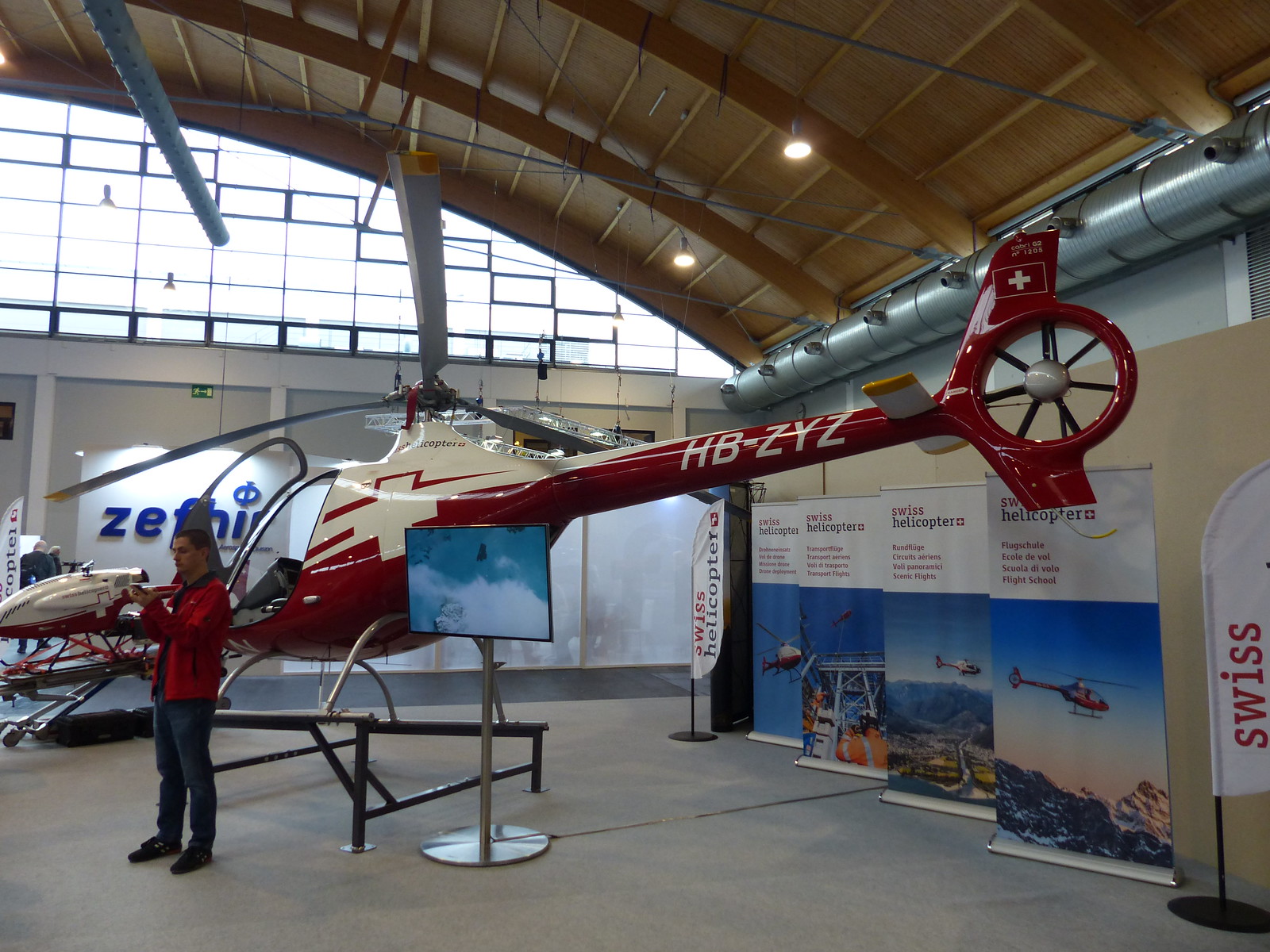The image depicts a scene from what appears to be an aviation or helicopter museum, likely in Switzerland. It features a red and white model helicopter with the tail number HBZYZ and a Swiss cross symbol prominently displayed. The helicopter has a three-bladed main rotor and is part of an exhibit that includes various banners and posters detailing Swiss helicopters. Standing to the left of the helicopter is a man dressed in a red blazer, blue jeans, and black shoes. He has short black hair and is holding a smartphone, possibly capturing the scene or reading information. The setting includes a curved, light brown, wooden ceiling with a large window that lets in natural light, highlighting the aircraft. The background also reveals several signs and flags, emphasizing the Swiss aviation theme. The man might be presenting or simply visiting, engaging with the displayed helicopter.